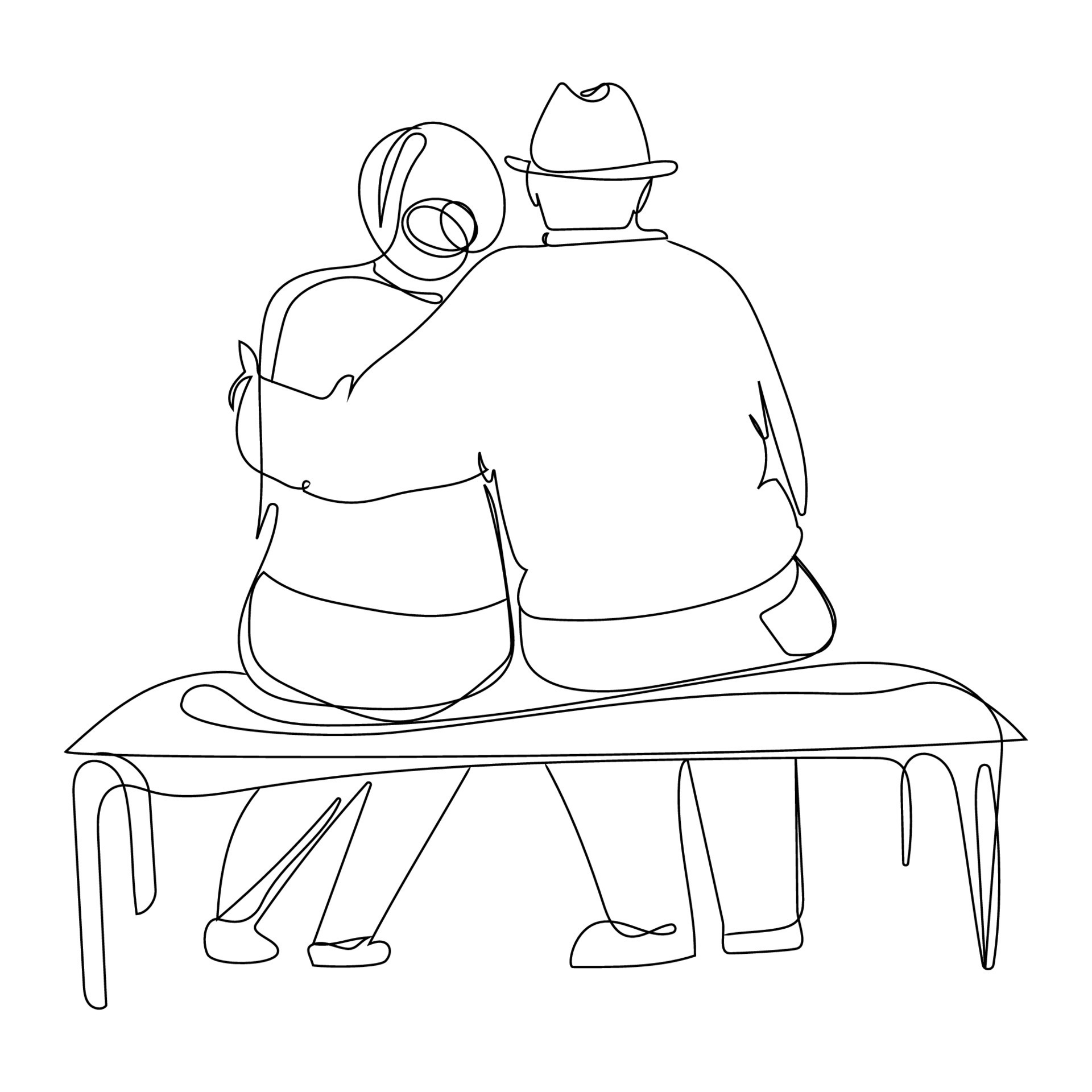This is a black and white line drawing illustrating an older couple sitting on a bench, depicted from behind. The style is reminiscent of John Lennon's simplistic line drawings, achieved without lifting the pen off the paper. The image consists solely of clean, continuous lines against a completely white background.

The woman, seated on the left, has her hair styled in a bun and wears pants and shoes. The man, situated to her right, dons a top hat, long-sleeved shirt, and pants. He is leaning towards the woman with his left arm wrapped around her shoulders, while she reciprocates by leaning into him. Notable details include the pocket line of the man's right hand on the back of his pants and the outline of a long bench they are seated on. The drawing captures the intimate simplicity and connection of the couple through minimalistic yet expressive lines.